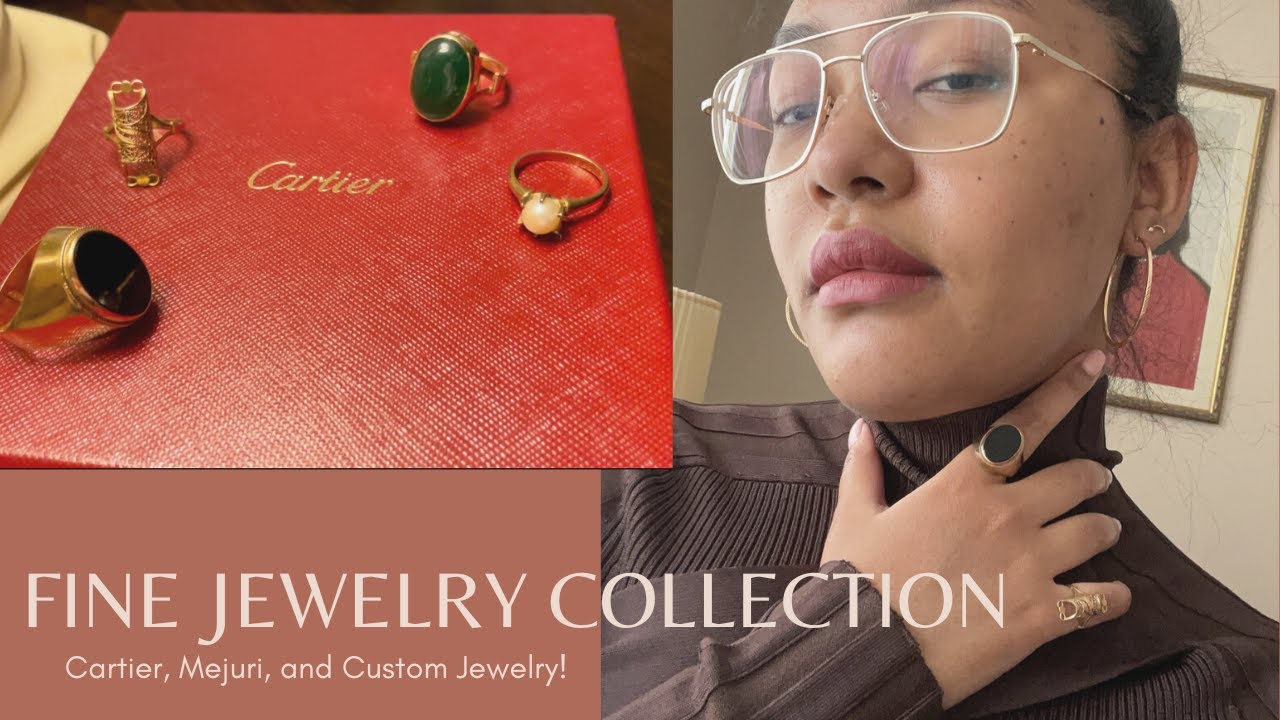The artwork is a detailed advertisement showcasing a Fine Jewelry Collection from Cartier, Mejuri, and Custom Jewelry, as indicated by the white text on the bottom left. The background is a soft rose color, enhancing the elegance of the image. In the top left, there is a red panel, likely made of vinyl, displaying the Cartier name in gold text, surrounded by several gold rings.

On the right side of the image, a woman serves as the model. She wears large, gold-plated wireframe glasses that highlight her face. Her lips are adorned with a subtle layer of lipstick or lip gloss. She is also wearing large round golden hoop earrings on both ears. Her outfit consists of a textured dark brown turtleneck, adding a touch of sophistication to her appearance.

The woman has two rings on her right hand; one is on her index finger, which is circular in shape, and the other is on her pinky finger. A gold-framed painting or portrait and a lamp with a cream lampshade provide a classic backdrop behind her, complementing the luxurious theme of the advertisement.